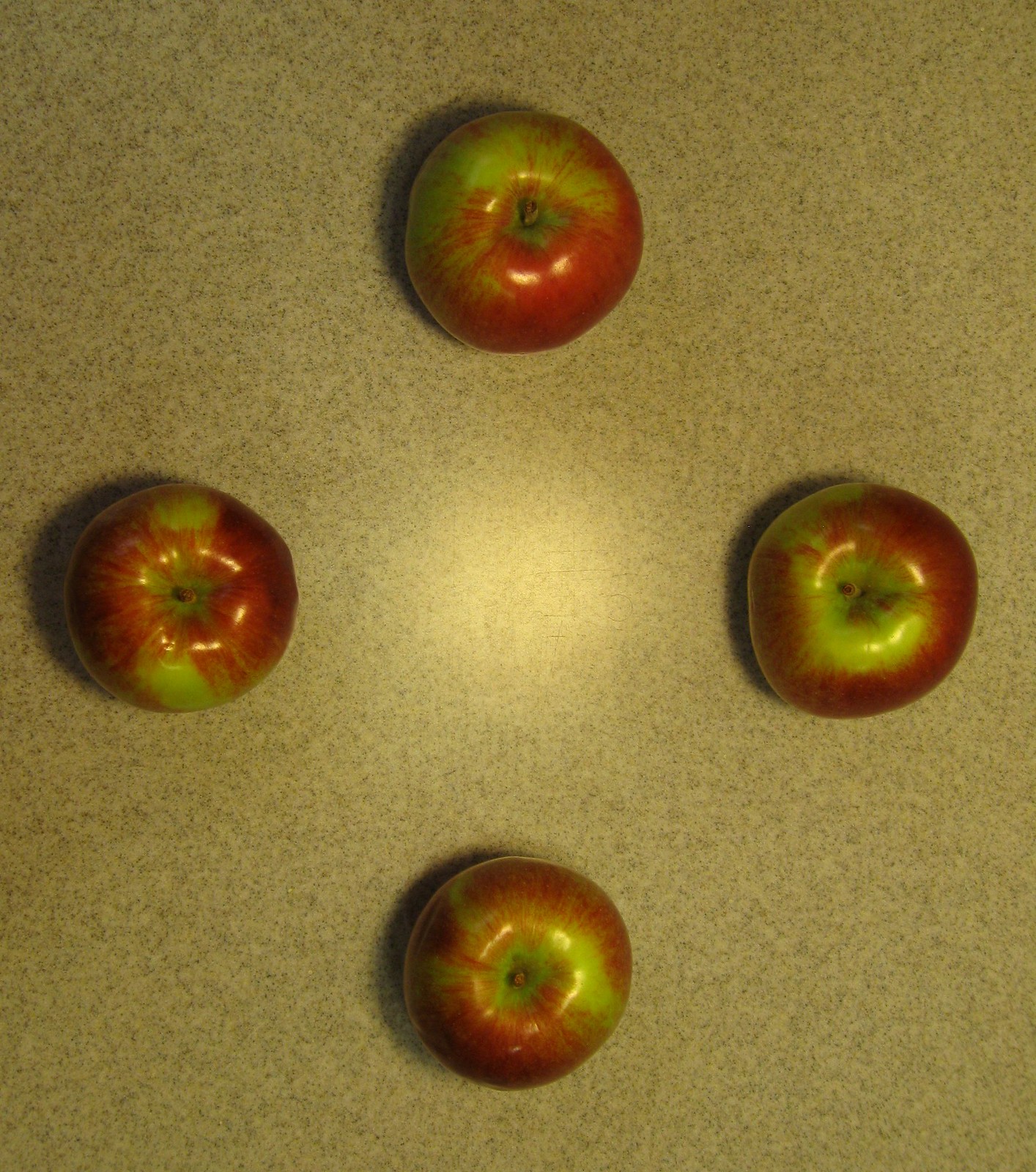This image depicts four shiny apples, each predominantly red with green patches, arranged in a precise manner reminiscent of a compass. They are placed in a square formation, representing the cardinal directions: north, south, east, and west. The apples lie on a golden-brown, marble-like surface, which suggests a kitchen countertop. The photo is taken from an aerial perspective, emphasizing the deliberate positioning of the apples. Depending on the viewer's orientation, the arrangement can appear as a diamond or a square. The smooth, reflective surface of the apples adds to their striking visual appeal in this meticulously composed scene.